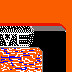The image appears to be a small, somewhat unclear screenshot, possibly from a video game. The dominant color is a vibrant, reddish-orange background. Below this, there is a black border. In the top-left section of the border, the letters "V" and "E" are displayed in white text, surrounded by small white dots that create a dotted border around the letters. Below this, the image resembles the edge of a TV screen, showcasing a chaotic mix of colors, including blue, green, white, and orange, arranged in a glitchy, pixelated pattern.